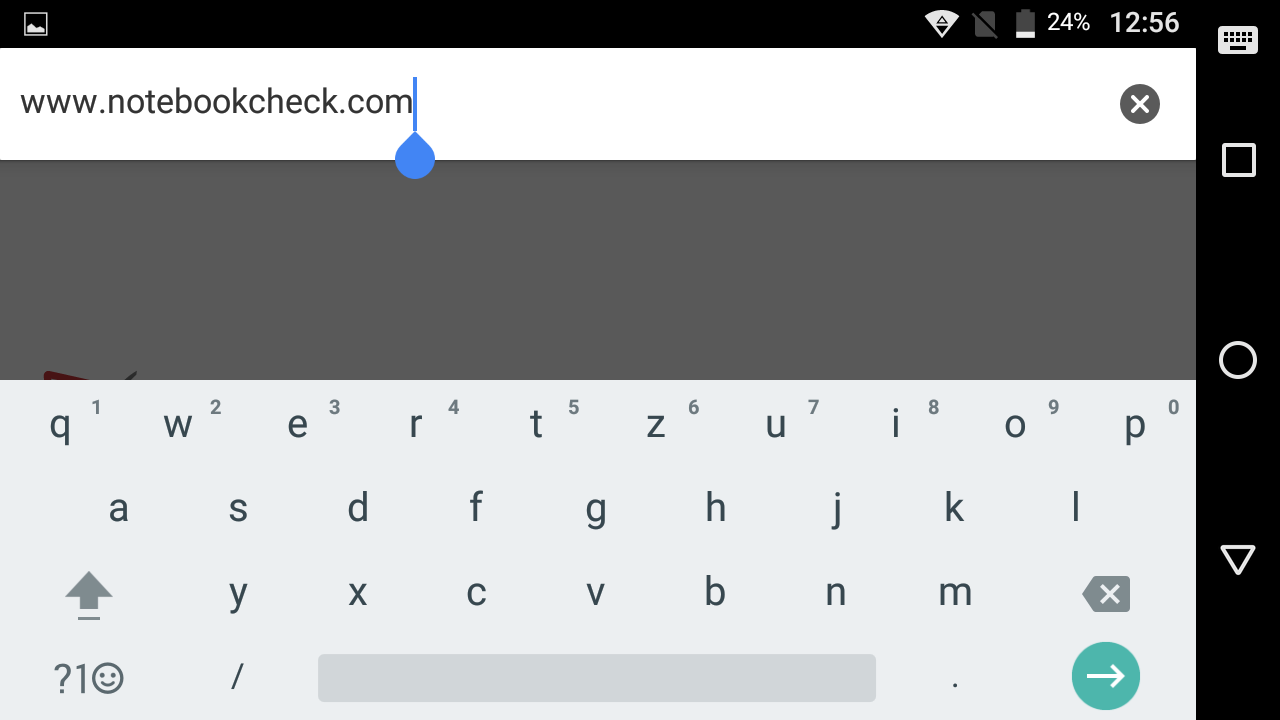The image captures a side-perspective view of a smartphone screen, featuring a web browser interface with an on-screen keyboard actively typing a web address. At the top of the screen, there is a black banner displaying several icons: a picture icon, a fully-filled Wi-Fi signal indicator, an icon resembling a sieve with a line through it, a battery icon at 24% charge, and a clock showing the time as 12:56.

Below this black banner, the web address bar shows "www.notebookcheck.com" with a blinking cursor and a blue text selection marker. Adjacent to the address bar on the right side is a circular icon with an "X" through it.

A gray banner separates the web address bar from the keyboard. The visible portion of the keyboard starts with the row containing the letters 'Q' through 'P', followed by a second row with 'A' through 'L', and the third row with 'Y' through 'M'. Below the letter keys, part of the space bar is visible, next to a green circular icon with a right-facing arrow.

At the bottom right corner of the screen, another black banner can be seen, featuring navigation icons typically found on smartphones: a square, circle, and triangle, symbolizing recent apps, home, and back functions respectively.

Overall, the image vividly captures a snapshot of a web browsing session on a smartphone, showcasing the user interface and functional elements in detail.